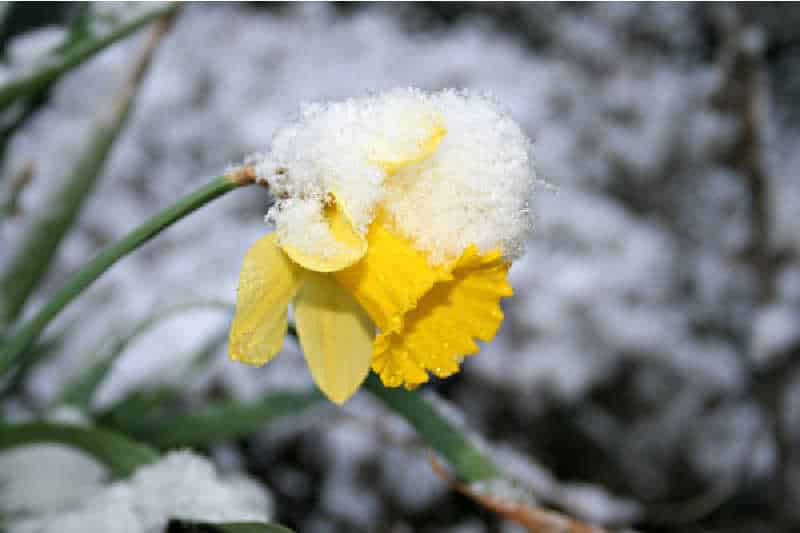The photograph captures a vibrant yellow daffodil on a green stem, prominently standing out against a blurred background. The scene is set outdoors, as indicated by the freshly fallen snow that blankets the ground. The daffodil, slightly leaning to the right, displays a trumpet-shaped central part and several additional petals beneath it. The flower's vibrant color contrasts sharply with a clump of snow that rests on its petals, possibly weighing it down and suggesting it's not in the best health. Additional green foliage can be seen jutting out from the ground to the right and left of the daffodil. The entire image has a soft focus, making the daffodil the clear focal point amidst a snowy and vegetative backdrop.